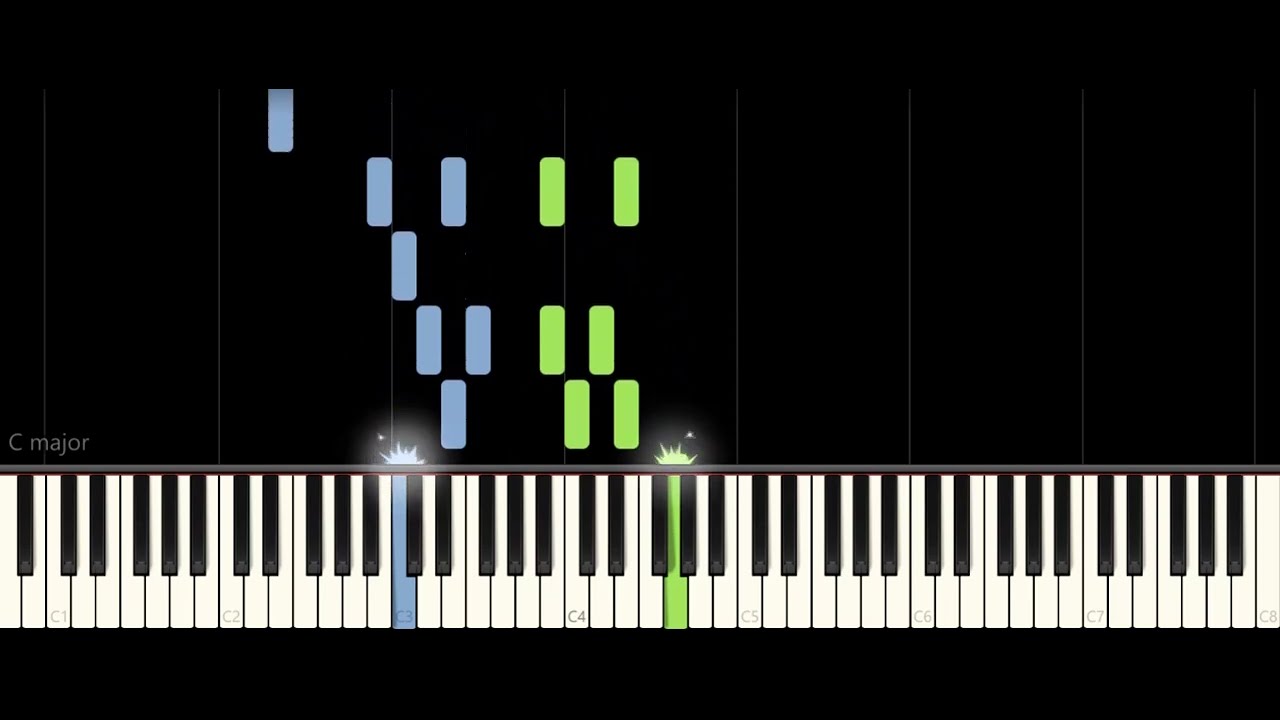This image showcases a virtual piano learning software viewed from above. Dominating the bottom portion of the image, the full length of the 88-key piano stretches across the frame, with keys visibly marked as C1 through C5 to denote octaves. The keys are in standard black and white, but a few stand out in blue and lime green, suggesting active notes. Above the keyboard, against a flat black background, are multiple rows of small rectangular tubes—seven blue and six lime green—indicating the notes to be played. Key presses are visually marked by an explosion-like logo, hinting at sound generation. In the top left corner, faded white text declares "C major," specifying the key signature in play. The design implies an interactive, step-by-step approach to learning or performing music through visual cues corresponding to the keyboard layout.